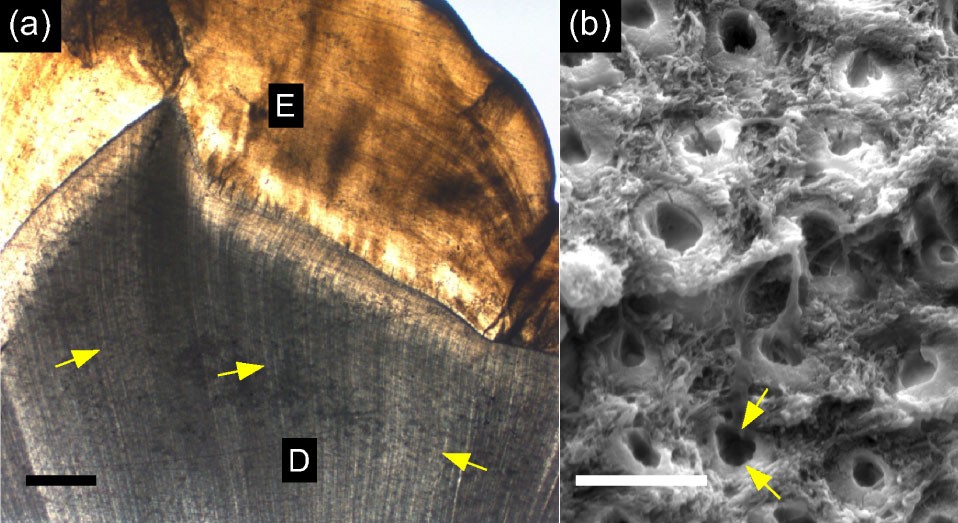This image features two detailed micrograph photographs, labeled A and B. The left photograph, A, showcases a close-up of a tree trunk cross section. The trunk is primarily marked by a gray vertical striated pattern labeled D, and a light brown top edge with a burnt appearance labeled E. The sections are demarcated with yellow arrows – two pointing from the left across the striated pattern and one arrow pointing from the right. This photograph also contains black squares indicating the labels A, E, and D, with a distinctive mountain-like shape at the base comprising vertical lines.

The right photograph, B, depicts a porous, foamy white substance bearing craters, presented in black and white. The texture in this image resembles wax or coral and is labeled with a black square marked B. At the bottom, two yellow arrows direct attention to one specific crater within the substance. These images, likely taken under a microscope and possibly from a textbook, detail intricate textures and patterns for observational purposes.